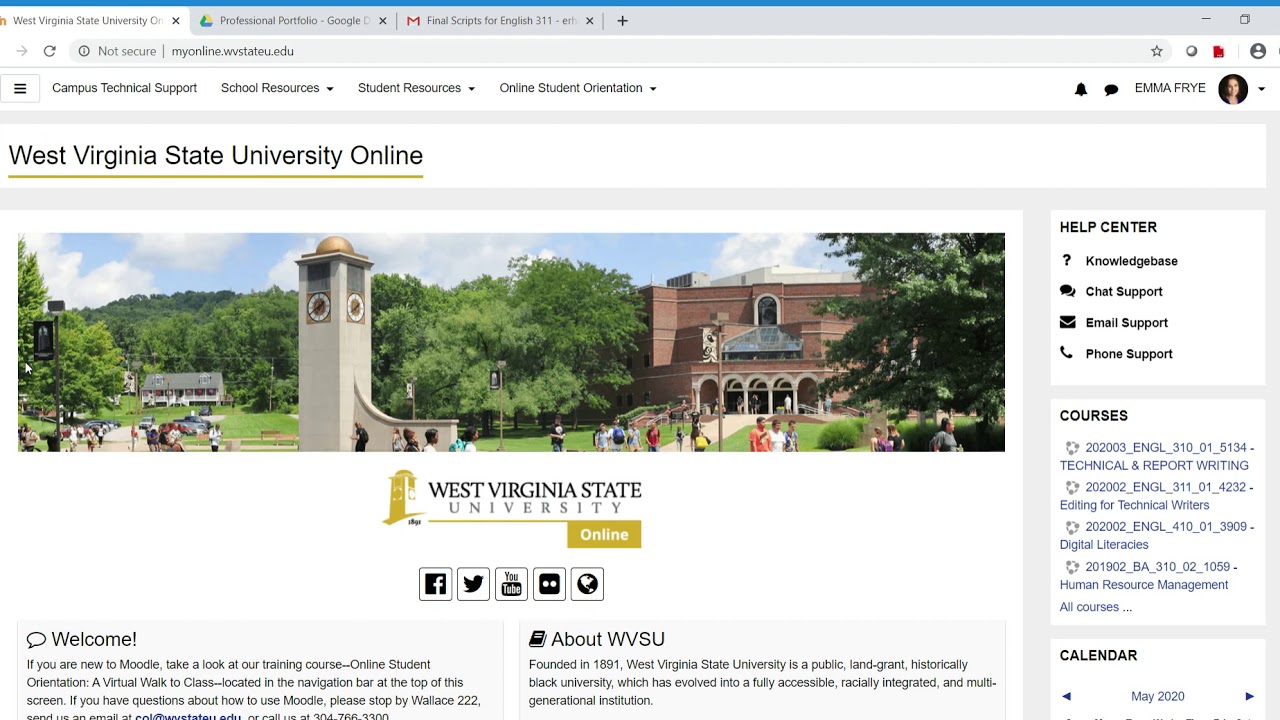The browser tab displays "West Virginia State University" with the URL "non-secure myonline.wvstateu.edu" underneath it. On the left-hand side of the page, there is a menu icon featuring three horizontal bars. Moving to the right, the navigation bar includes "Campus Technical Support," "School Resources" with a drop-down menu, "Student Resources" with a drop-down menu, "Online Student Orientation" with a drop-down menu, and icons for profile settings, notifications (bell icon), messaging (speech bubble icon), and the user profile for "Emma Frye," indicated by a circular profile picture of a white girl with dark hair and her name spelled as "Emma Frye."

Below the navigation bar, the main content starts with the header "West Virginia State University Online," accompanied by a photograph of the university. Directly below this image is a logo-like representation of "West Virginia State University Online," with the word "Online" styled to resemble a button in mustard yellow, white, and black colors.

Scrolling further, there are social media icons for Facebook, Twitter, YouTube, a square with two dots (possibly Instagram), and a globe icon (possibly indicating international resources or global navigation). A welcoming section reads: "Welcome! If you are new to Moodle, take a look at our training course online."

This detailed description captures the layout and elements of the webpage, providing a comprehensive understanding of the visual and functional components present.